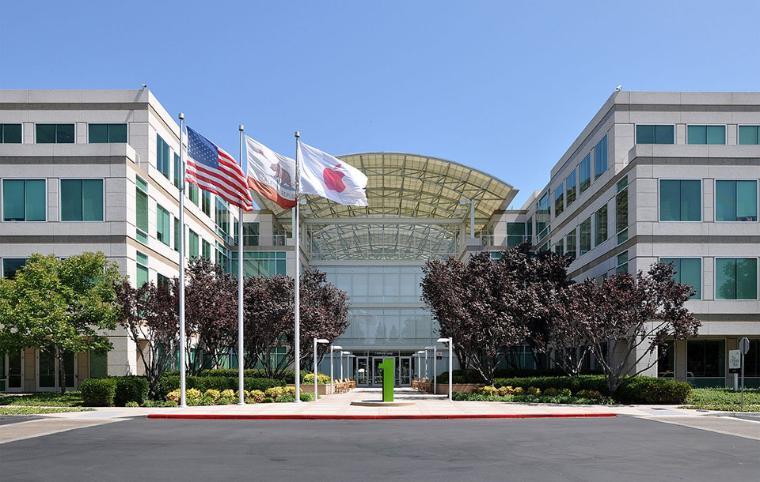This image depicts the front of an office building complex, likely the Apple headquarters, featuring a prominent glass awning and a central walkway flanked by symmetrical square buildings on either side. In the center of the walkway, there is a green rectangular vertical monument. Three flags are positioned to the left: the American flag on the very left, the California state flag with a bear in the center, and the Apple logo flag to the right. The walkway is lined with landscaping elements, including a green tree to the far left, two maroon-leafed trees on each side, and several shrubs. Other notable details include lights along the walkway, some seating areas, and security cameras atop the building. The building itself has numerous glass windows and appears to be primarily constructed of concrete. An amphitheater-style awning covers the main entrance lobby, which is recessed from the courtyard. There is a stop sign to the far right of the image, indicating the presence of nearby roadways. The setting is during the daytime under a clear blue sky, with no visible people in the scene.